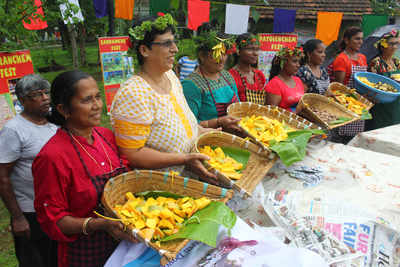This photograph captures a vibrant scene at what appears to be a competition or fair, featuring a group of eight women and one man. The women, some of whom are adorned with leafy wreaths and flower crowns, hold up baskets containing bright yellow items, possibly cut fruits. They are all looking intently toward something off-camera to the left, their expressions suggesting focus and anticipation. The man in the background, wearing a gray shirt, stands slightly behind them, also gazing in the same direction. In front of the participants, a table covered with crumpled newspaper hints at the activity's nature—perhaps some form of preparation or display. The setting is festive, with a string of solid-colored flags in green, orange, blue, white, and red hanging behind them. This lively tableau suggests a communal event celebrating cultural or agricultural prowess, possibly among Islander communities.